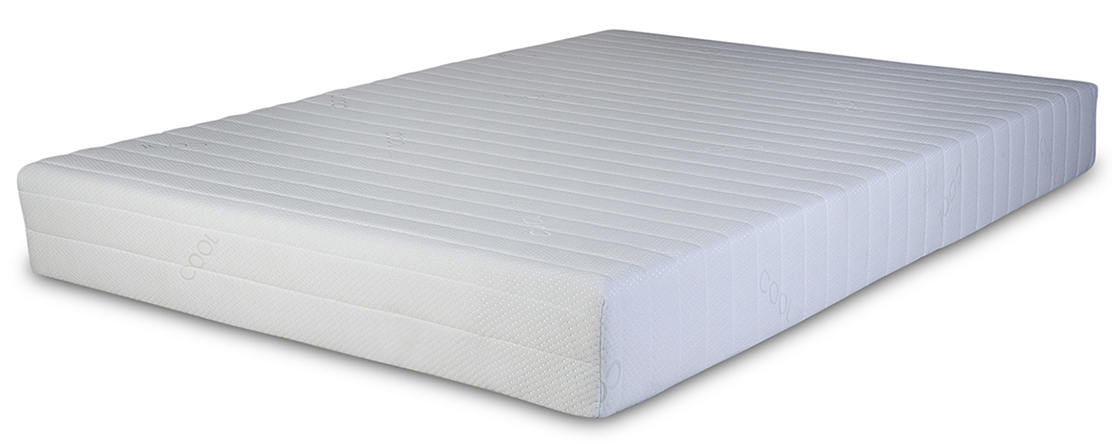The image features a large, low-profile king-size mattress laying flat on a completely white background, positioned diagonally in the center. The mattress itself is off-white with shades of grey and some light blue hues, varying depending on how the light strikes it. The perspective shows multiple angles: the top, the base, and the right side of the mattress, revealing a ribbed pattern with detailed stitching. Unlike the rest of the mattress, the top front features two straight lines of stitching and includes a visible piece of text that says "Cool!" The image appears to be taken in a style typical for a mattress retailer's website display, and there is no additional text or objects other than the mattress and possibly a watermark.